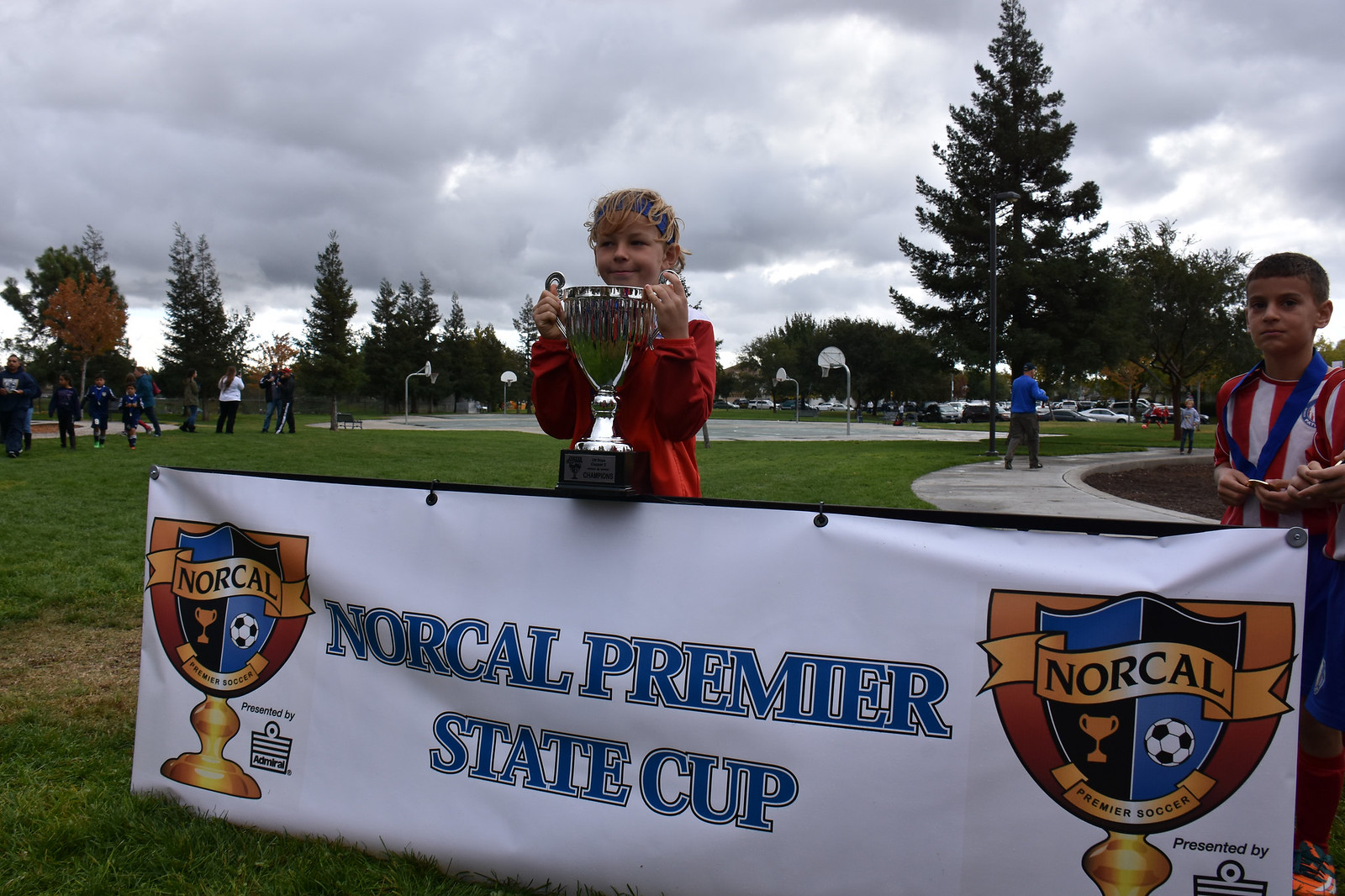In the center of the image, a smiling boy wearing a red long-sleeve shirt proudly holds up a large trophy. To the right, another child in a red and white striped shirt stands. The bright, daytime setting is evident despite the cloudy sky. Behind the children, people casually stand around, and lush green trees and parked cars are visible, creating a lively atmosphere. A prominent banner at the bottom of the image reads "NorCal Premier State Cup," flanked by animated images of trophies and a soccer ball. The vivid, colorful image captures a joyful moment at the NorCal Premier Soccer event.